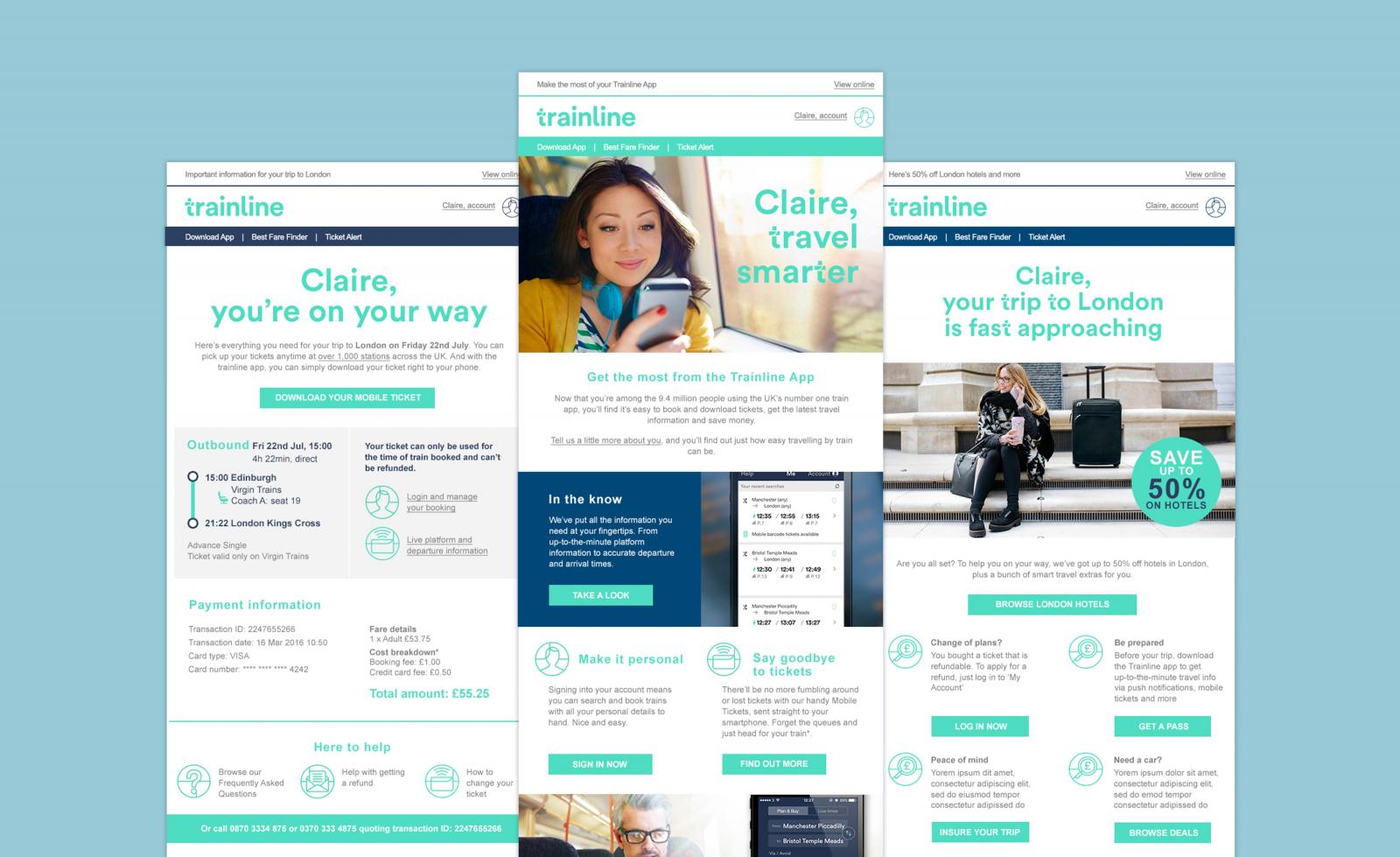The image is a composite of three screenshots from the same website, each showcasing different content related to travel. 

The middle screenshot prominently features the title "Train Line" in green text at the top left. Below this title is a photograph of an Asian woman with brown hair, glancing at her silver-colored phone. She wears headphones around her neck, sports a yellow jacket over a white and green blouse, and has her nails painted red. To the right of her photo, the text reads, "Claire, travel smarter."

The right screenshot also has "Train Line" at the top left. At the top center, it says "Claire, your trip to London is fast approaching." The image features a different woman, sitting on some stairs, with her briefcase placed to her left and her purse in her hands. She is dressed in an all-black outfit.

The left screenshot shows "Train Line" again at the top left. In the middle left section, it states, "Claire, you're on your way." Below this text, there is a grayed-out box showing the address "1505 Edithsburg" and mentioning a trip to London.